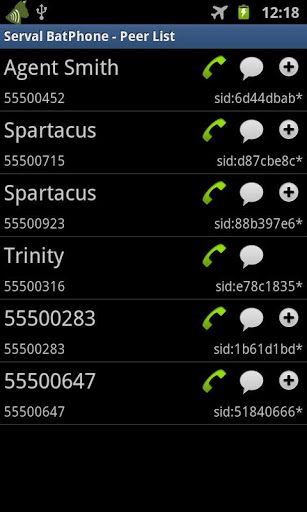This image captures a phone screen displaying a contacts list. At the top of the screen, icons depict a bowl, a cactus, and an airplane. The battery icon is green, indicating a healthy charge, and the time displayed is 12:18. On the left side, the heading reads "Servo Bat Phone". Below are columns labeled "Peer List" and "Agent Smith" accompanied by a phone number. Icons for phone calls, text messages, and an additional option follow. The name "Spartacus" appears twice, each entry with a different phone number. Further down, the name "Trinity" is listed along with the phone number 555-00283. Another contact below displays the number 555-00647. All entries include icons for making a phone call, sending a message, and an additional option.